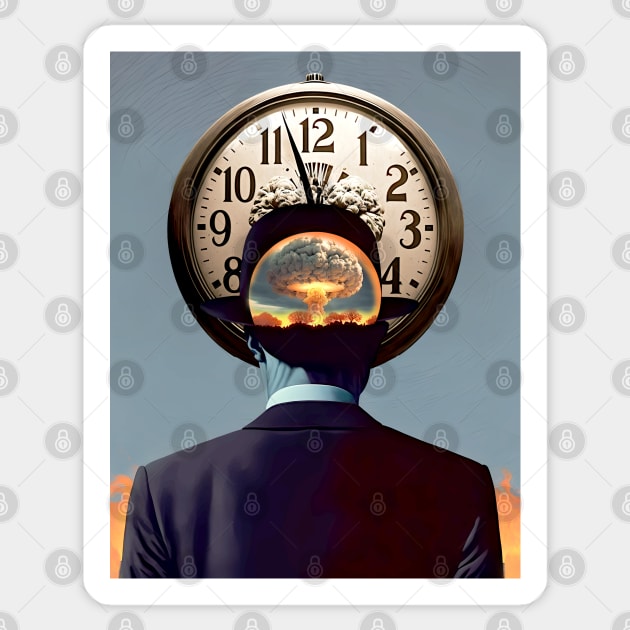The image is a dynamic and abstract visual artwork blending elements of photography and illustration. At its core, the image features a monochrome photograph of a man seen from behind, prominently dressed in a black suit and white shirt, topped with a black cowboy hat. The man faces away from the viewer, directed towards a large, circular wall clock with a dark-brown bezel and a white face, its black hands nearly striking the 12. Intriguingly, an image of a nuclear explosion is superimposed on the back of the man's head, with a mushroom cloud of orange and yellow flames extending outward, seamlessly melding into the scene. Adding to the surreal atmosphere, the man appears amid scattered lock symbols across a blue-gray background, underscoring themes of time, security, and impending doom. The entire composition, reminiscent of a playing card’s design, suggests a dramatic countdown, echoed by the "doomsday clock" concept with only 90 seconds remaining to an implied cataclysm.